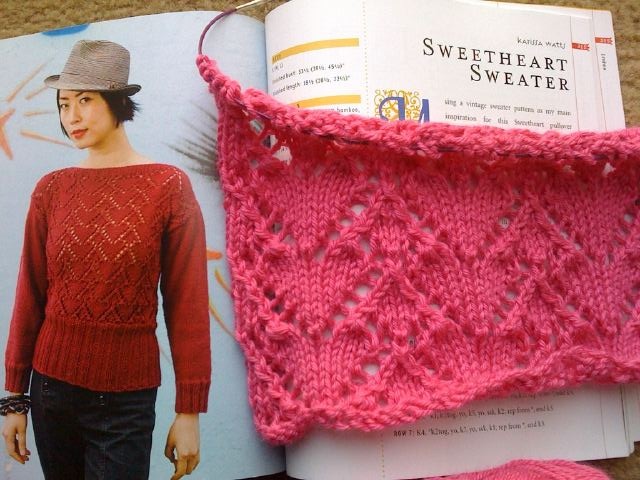In this image, an open book titled "Sweetheart Sweater" showcases a detailed knitting pattern for a heart-patterned sweater. On the left page, a model is seen wearing the completed sweater, which is a deep fuchsia pink and features a subtle heart motif created with see-through holes in the knit. The model, with short black hair, is dressed in black slacks, a gray fedora, and has a bracelet on her right wrist. Her arms rest naturally by her sides as she stands against a seemingly superimposed background of the open book. Surrounding the knitting instructions on the right page, a partially completed bright pink knitted piece encircles the text, still attached to the knitting needles, demonstrating the pattern in progress. The yarn's support thread is visible, indicating the work is not yet finished. The vibrant pink material obscures much of the text on the page, leaving only parts of the "Sweetheart Sweater" title and minimal other writings legible. The overall scene blends the stages of creation with the finished product, vividly depicting the journey from pattern to final garment.